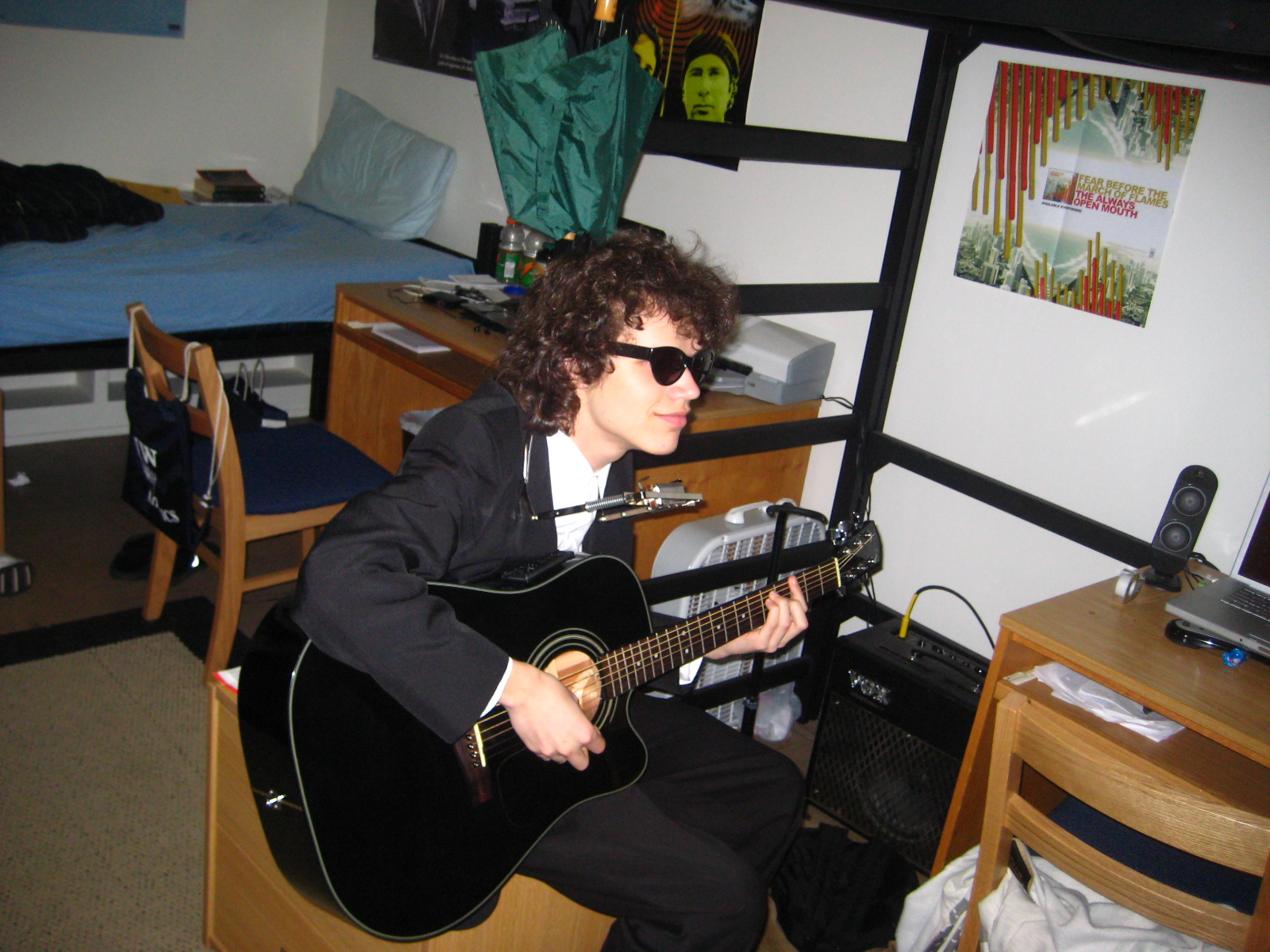The image depicts an indoor setting, likely a cluttered bedroom, featuring a young white male seated atop a wooden stand. He has mid-length curly brown hair and wears dark black shades, a white top, a black jacket, and black trousers. The man is engaged in playing a black guitar, which is plugged into an amplifier located behind him. In front of him, to his right, there's a corner of a laptop and a webcam set on a small desk, along with a roll of sellotape. Behind him, the unmade bed is visible with a pillow and a bedside table that holds a book. A brown desk with a chair in front of it occupies the background, alongside a white box fan on the floor. The walls of the room are all white, and next to the desk at the lower right, there are additional speakers and another small desk.